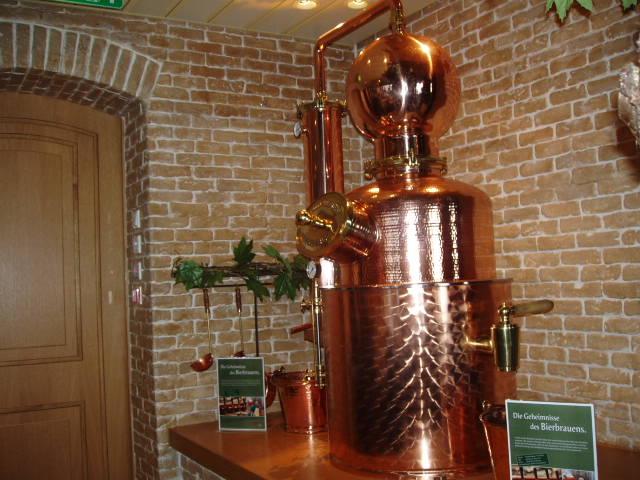The image depicts a highly polished, large, old copper urn with a shiny, reflective surface, sitting on a table in a room with a brick wall and a brown door to the left. The urn, which has a rounded top and a glassy appearance, features a spigot with a handle control on the right-hand side and a copper pipe that enters a bulb on its upper part, connecting to other piping, possibly for distillery purposes. On the urn, there are pressure meters. A small bucket is positioned behind the urn to the left, and there are two unreadable signs on either side of it. Light is flowing onto the urn, enhancing its gleaming surface. The setting and elaborate features suggest it's more of an ancient, display piece rather than a functional coffee urn.